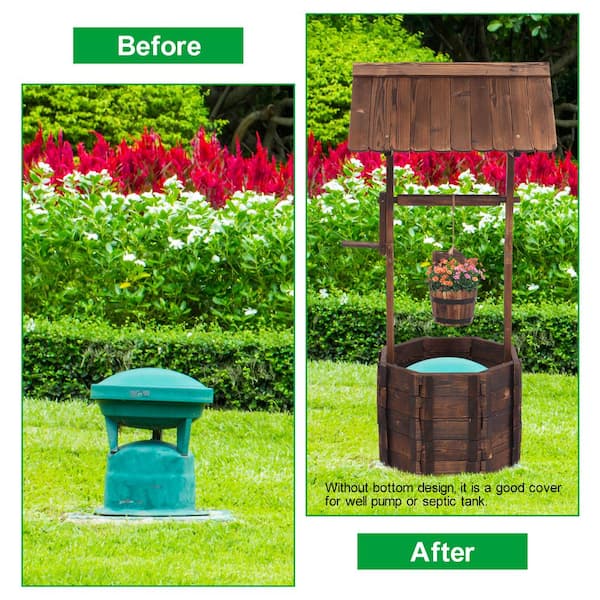This two-part image shows a before-and-after comparison of a backyard landscape, likely for marketing purposes. The left side, labeled "BEFORE" in a green bar, displays a garden with a well-maintained lawn, hedge, and colorful flowers. In the grass sits an exposed blue-green cylindrical object, possibly a well pump or septic tank cover, on a small concrete platform. The right side, marked "AFTER" in a green bar at the bottom, reveals the same garden with a decorative wooden structure elegantly hiding the previously visible object. This wooden wishing well features a small roof, a hand crank, and a wooden bucket filled with pink flowers, mimicking an old-fashioned well. The design is intended to discreetly conceal plumbing elements, enhancing the aesthetic appeal of the backyard. In black text, it notes the well cover’s practicality: "Without bottom design, it’s a good cover for a well pump or septic tank."